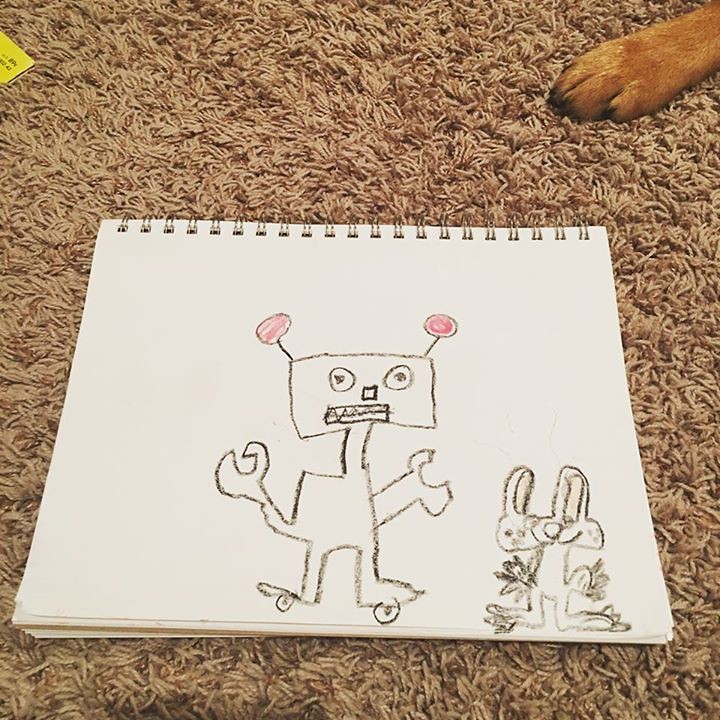An open sketchbook lays on a brown carpet, displaying a charming children's crayon drawing. On the blank white page, a robot and a peculiar two-faced bunny are illustrated with thick black crayon lines. The robot, featuring a square head and body, wields wrench-like hands and rolls on wheel-like feet. Two tentacles with pink circles at their tips extend from the robot. Beside the robot stands the unusual bunny with a split head adorned with an ear on each side, a strange smile, and quirky eyes. In the upper right-hand corner of the sketchbook, a brown dog's paw is visible, as if the dog is observing this whimsical artwork.